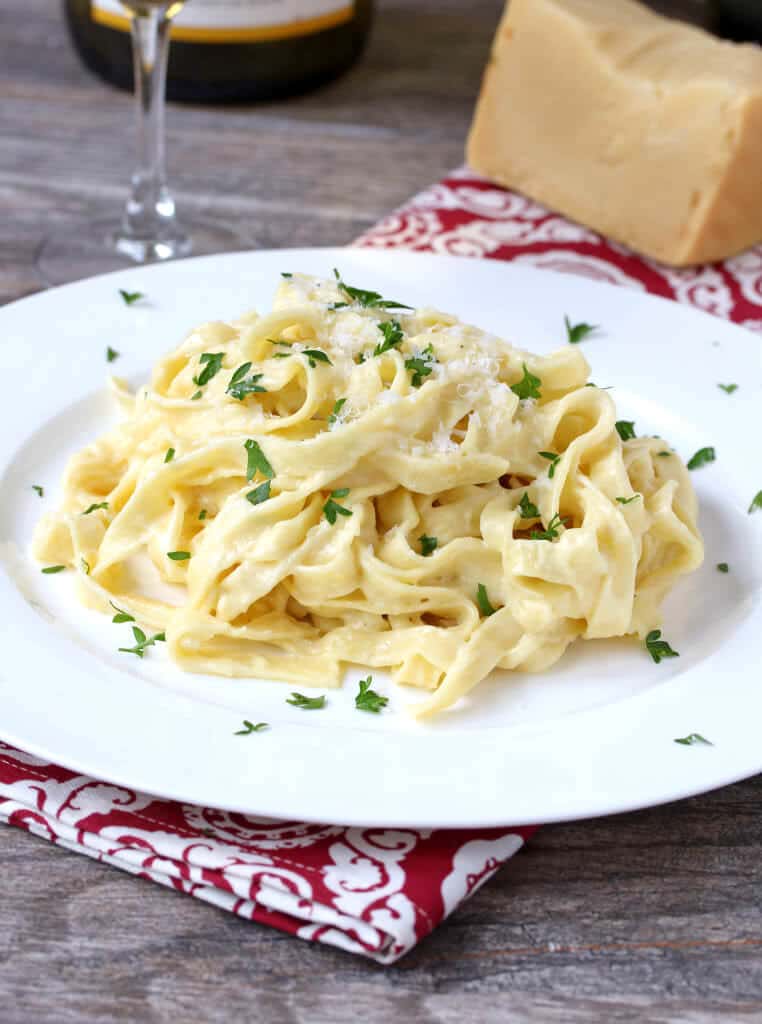This detailed close-up food portrait showcases a beautifully presented plate of freshly prepared fettuccine alfredo. The fettuccine noodles, covered in a rich, creamy alfredo sauce, are artistically swirled and mounded on a white ceramic plate with a central indentation. Generous shavings of parmesan cheese and a sprinkle of finely chopped parsley or cilantro adorn the top of the pasta, and additional green herb bits are scattered around the plate's edges.

The white plate is placed on a folded red and white floral-patterned napkin, which adds a touch of elegance and contrast to the presentation. This ensemble rests on an ash gray, wood-grain textured tabletop that provides a subtle, rustic background.

In the background, towards the upper right, a partially grated block of parmesan cheese sits on the napkin, indicating the freshness of the ingredients. To the top left, the slender stem of a wine glass is visible, accompanied by the base of a dark-colored wine bottle with a white label trimmed in yellow, hinting at a sophisticated dining ambiance. The overall composition highlights the richly textured and creamy pasta, enhanced by the thoughtful garnishments and harmonious color palette of the setting.